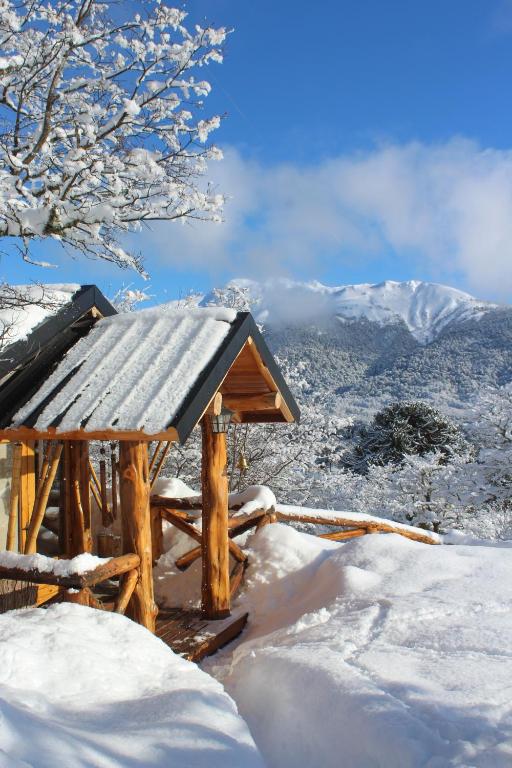A full-color vertical photograph captures a serene winter scene outdoors, showcasing a cozy wooden cabin nestled in a mountainous, highly elevated region. The clear blue sky, adorned with sparse white clouds, provides a stunning backdrop. Just below the cloud line runs a snow-covered mountain range, emphasizing the cabin's lofty position. The cabin, situated in the center-left of the image, features traditional wooden construction with a green, metal pointed roof partially blanketed in snow. At the top left corner, a snow-covered tree extends its bare branches over the cabin, adding to the wintry charm. The structure's entrance, framed by golden-yellow logs and topped with the metal roof, remains prominent, flanked by a deep snow pathway that meanders from the entrance to the lower right-hand corner. The snow in the forefront is deep, at least three feet high, surrounding the pathway. Additional snow-covered trees punctuate the background, with one appearing distinctly greener than the others, contrasting against the pervasive whiteness. The scene encapsulates the tranquil beauty of a wintery mountain retreat.